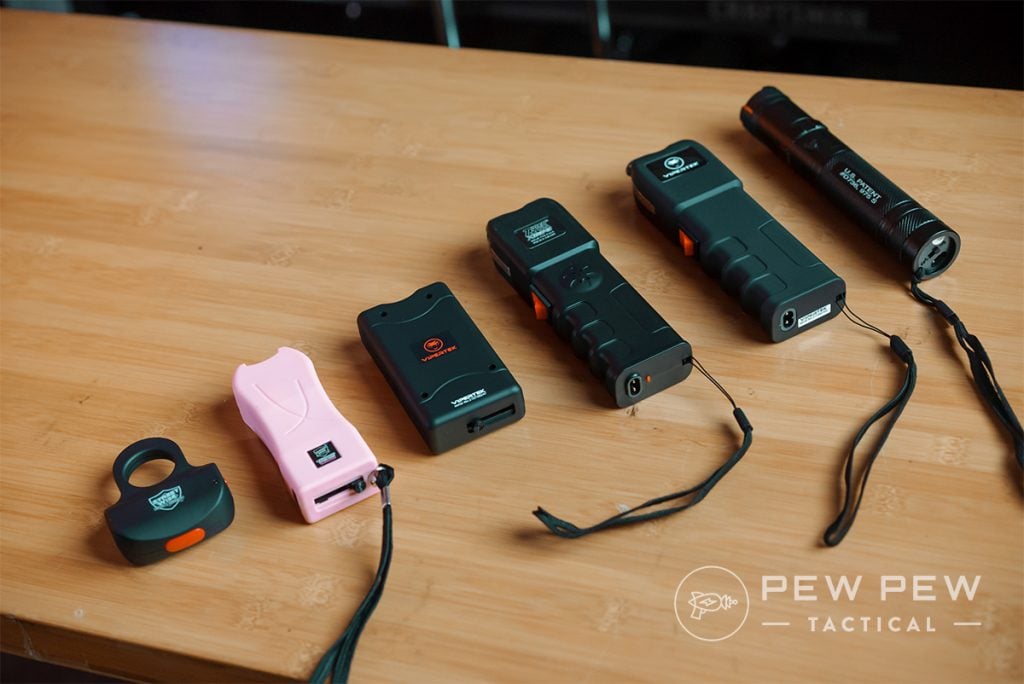In this detailed photograph, six different tasers are meticulously arranged on a light brown wooden table, commonly found in school settings. Starting from the bottom left, the first taser is a small black unit with a central hole large enough for one or two fingers, featuring a flared bottom, a green logo in the middle, and a red button. The second taser is pink and rectangular, equipped with a black cord loop for wrist attachment and some black writing at the bottom. The third taser is also black and rectangular with red writing on the top. The fourth device is a longer black taser, segmented into two sections with a red side button, white text at the top, and a wrist strap. Similarly, the fifth taser matches the fourth but includes a white sticker at the bottom. The sixth device is distinctively cylindrical and resembles a flashlight, marked with white writing and accompanied by a wrist strap. All tasers are evenly spaced and slanted towards the bottom right of the image. In the bottom left corner, there is white text reading "Pew Pew Tactical" next to a circular logo depicting a gun.